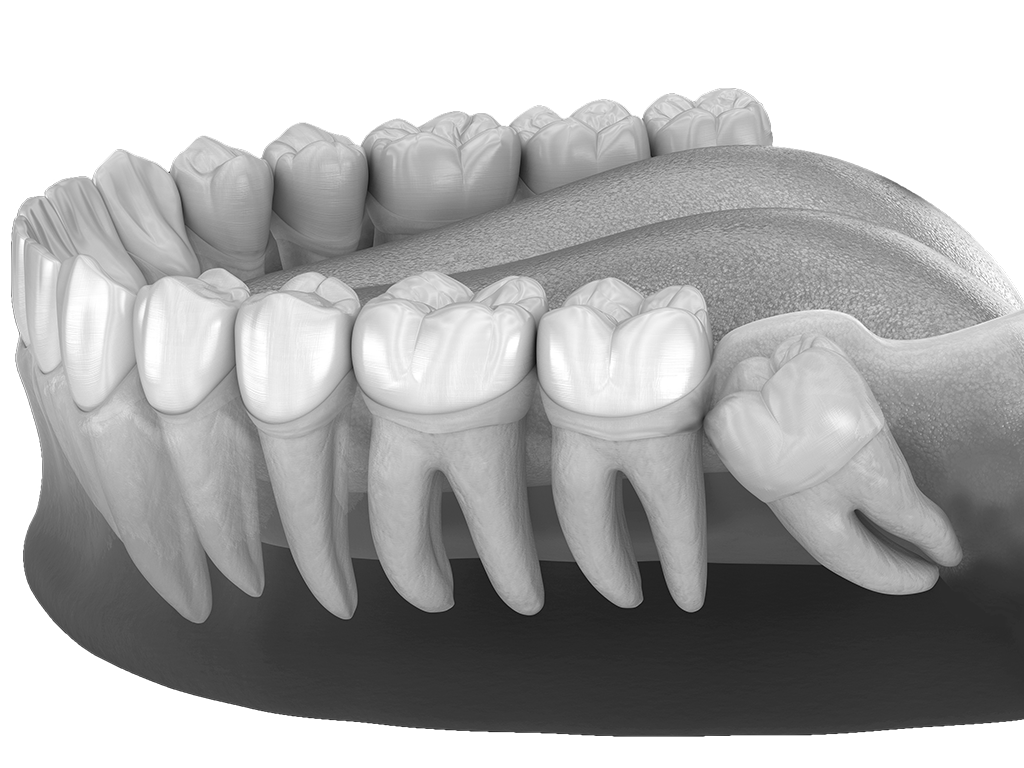This detailed black and white digital diagram showcases a full set of healthy lower teeth, emphasizing their well-maintained enamel and straight alignment. Highlighted in the image is a single impacted wisdom tooth on the left side at the very back, which is noticeably slanted backward due to its crooked root. Unlike the pristine, white-toned teeth with visible roots extending into the gums, this wisdom tooth disrupts the otherwise orderly dental arrangement. The backdrop of the image is entirely black, accentuating the grayscale display of the teeth and roots, commonly used in dental visualizations for educational purposes.